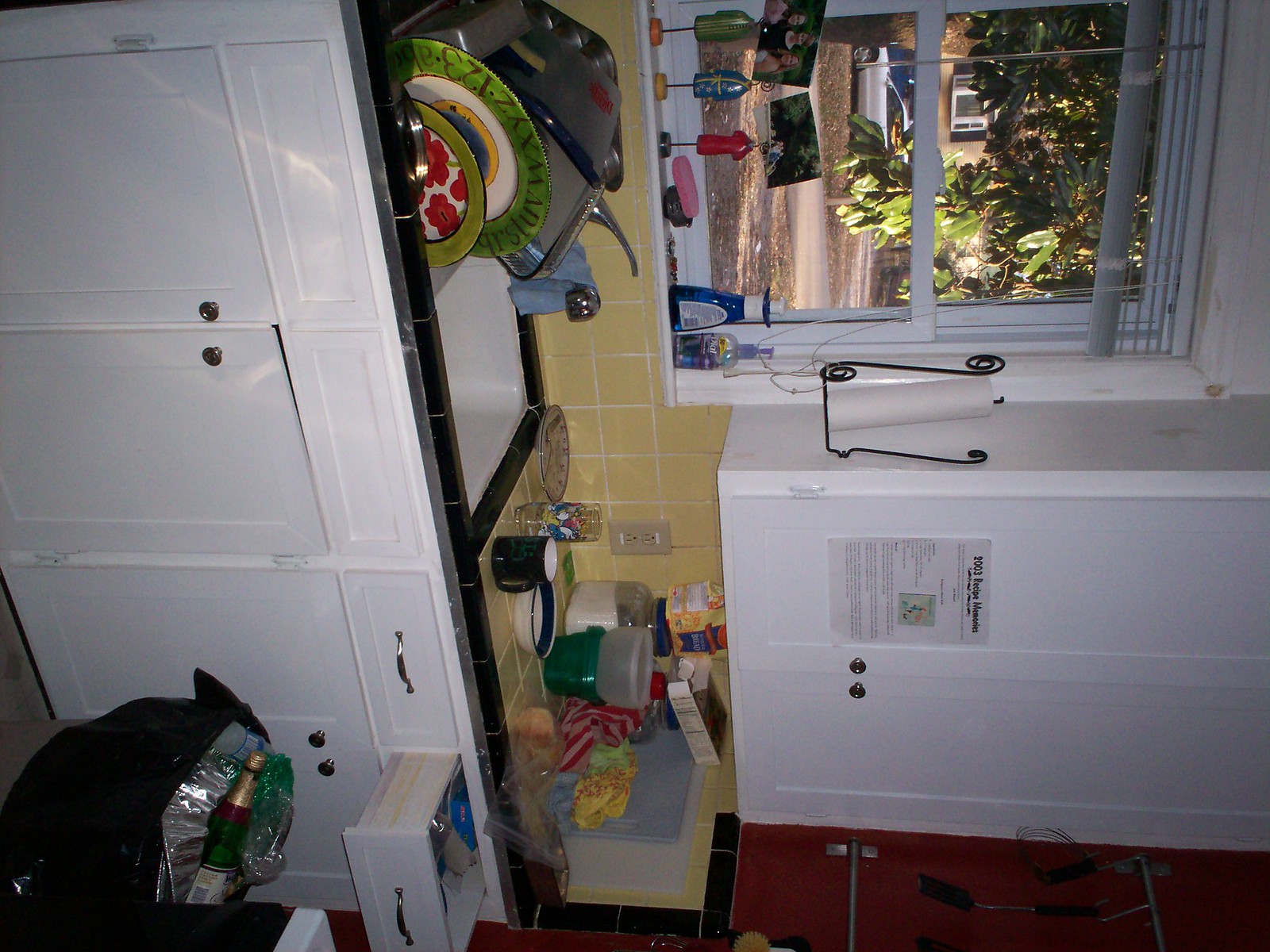This color photograph, taken in portrait mode and oriented sideways, captures a vibrant kitchen scene. Central to the image is a white wall cabinet with two silver knobs, prominently situated where the doors open. The upper door displays a white label with black printing. Adjacent to the cabinet, a black wrought iron paper towel holder is fixed to the wall, featuring intricate swirl designs at both the top and bottom.

An open window, dressed with white Venetian blinds pulled up at the top, allows a glimpse of a lush tree outside, possibly a magnolia, with its shiny, green, oval-shaped leaves in full display. The windowsill beneath showcases three colorful decorative items, each elegantly perched on wooden stands. Nearby, a bottle of blue dish soap and a clear bottle of hand soap stand ready for use.

The kitchen wall is adorned with yellow tiles, creating a warm backdrop for the sink area below. The countertop is composed of black tiles, adding a striking contrast. On the left side of the sink, dishes are stacked, while the right side of the counter is cluttered with various items. Below, an open drawer reveals the silver-colored handles and knobs of a white base cabinet. On the floor, an open black plastic garbage bag contains what appears to be a champagne bottle and a silver foil pan. This detailed snapshot of a kitchen offers a peek into an everyday, yet character-filled, domestic space.